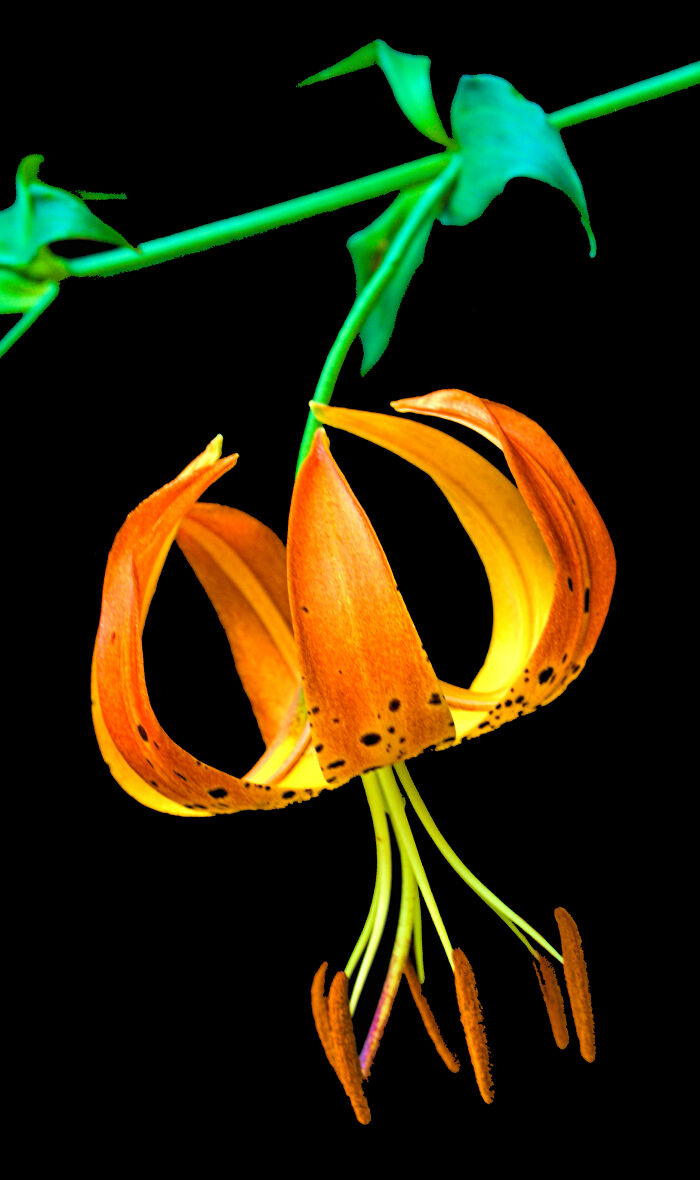This detailed color photograph showcases an exotic tropical lily in full bloom, captured in portrait orientation against a solid black background. The vibrant flower hangs upside down from a bright, vivid green stem that leads to a cluster of slender green leaves, slightly tilted to the left. The striking petals of the lily, primarily orange with hints of red at the tips, gracefully curl upward and exhibit distinctive black speckles near their bases. The undersides of the petals reveal a pale yellow hue accented with red ribbing. Emerging from the center of the blossom, several yellow stamen adorned with elliptical brown seeds extend downward, their fine brown pollen giving them a fuzzy appearance. This image exemplifies photographic representationalism realism, providing a captivating and highly detailed view of the flower's intricate beauty.